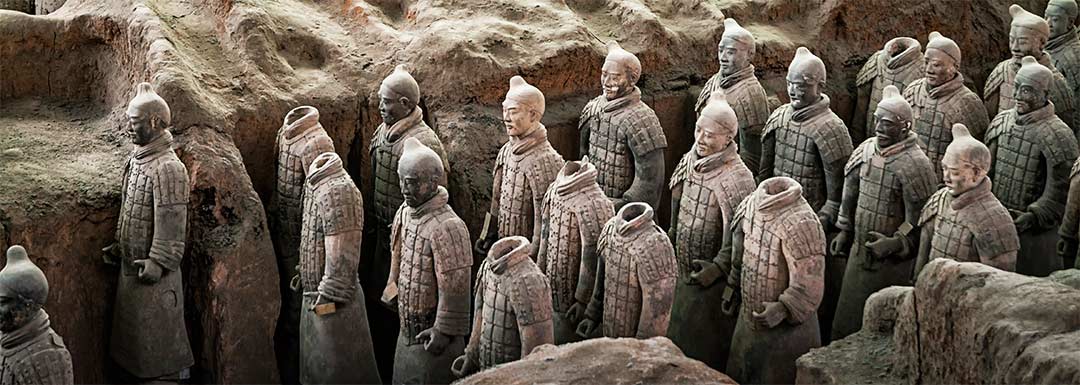The photograph captures an outdoor excavation site displaying the ancient Chinese Terracotta Warriots statues. The image reveals a row of these meticulously crafted clay soldiers standing in unison, donned in identical or nearly identical military attire, characterized by detailed armor, ridge-patterned shirts, and top knots. Some statues are missing their heads, leaving behind empty neck holes, while others remain intact. Interestingly, the statues exhibit a range of colors, some being carved from lighter rocks and others from darker materials, creating a striking contrast. The background features the textured, bumpy ledges of the excavation pit, highlighting the rugged terrain from which these historical artifacts were unearthed. This stone army, believed to be guarding the Emperor in the afterlife, faces left, epitomizing the silent vigilance they were designed to embody.